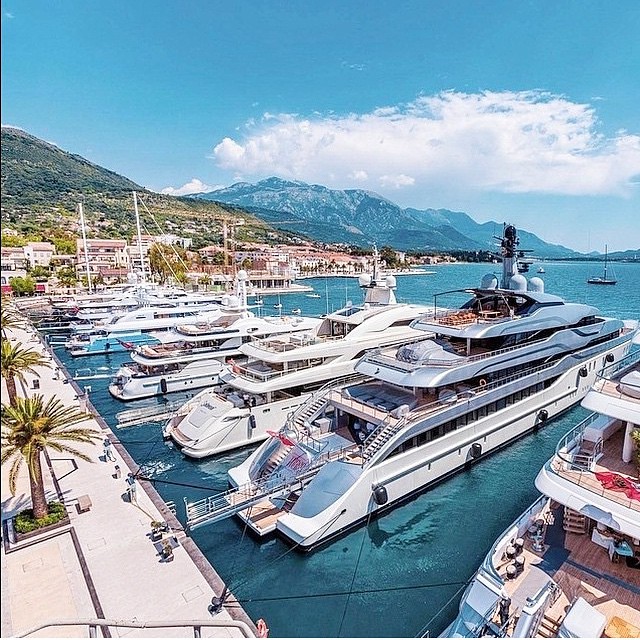This vibrant photo, reminiscent of a postcard from a tropical paradise, showcases a picturesque marina, possibly in the Caribbean or Mediterranean. Dominating the scene are six enormous, multi-level luxury yachts, each docked with a walkway extended for easy boarding. The yachts are nestled in crystal clear, turquoise waters that reflect the vessels like a glassy mirror, hinting at a nearby reef. Among these grand yachts, a smaller sailboat gently sails further out, accompanied by several other sailboats with visible masts.

On the left side of the image, a boardwalk lined with palm trees hints at the warm, inviting climate. In the distance, a quaint village with houses climbing the hillside adds a charming touch to the landscape, framed by towering mountains that extend down the waterway. The sky mirrors the water's clarity with a brilliant blue hue and is adorned with a single, large puffy cloud. This high-quality image, free of text, captures the serene yet vibrant essence of coastal luxury living, perfect for a travel promotional material or personal memento.